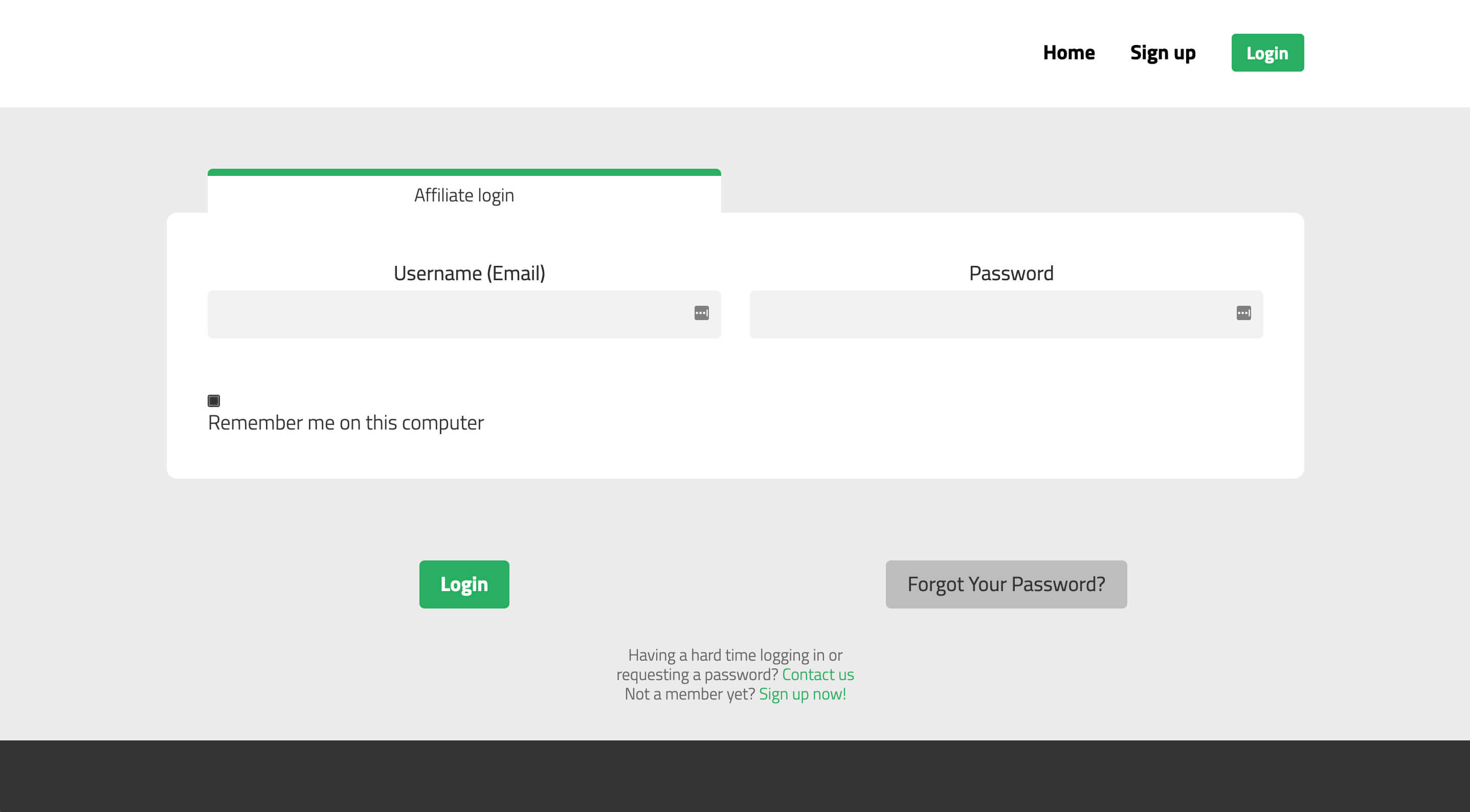The image depicts a login interface for an unidentified website. The layout is structured with a primary focus on affiliate login credentials.

In the top-right corner, there are navigation options: “Home,” “Sign Up,” and “Login.” The “Login” option is uniquely highlighted with a green box and white lettering.

The central portion of the interface prominently features an “Affiliate Login” section, denoted by a green banner that matches the “Login” button's color from the top-right corner. Directly below, there are fields labeled "Username (Email)" and "Password," each accompanied by a gray rectangular input box for entering the respective credentials.

Beneath these fields, there's a "Remember me on this computer" option marked by a black checkable square box. Adjacent to these elements, on a horizontal line, is a green “Login” button that seamlessly integrates visually with the affiliate login banner.

The entire affiliate login section, including the input fields and the "Remember me" checkbox, is enclosed within a white rectangular box, creating a distinct separation from the rest of the page.

At the bottom of this section, the interface provides additional support options: "Having a hard time logging in?" and “Forgot your password?”. For new users, it encourages account creation with messages like "Not a member yet?" followed by “Contact Us” and “Sign Up Now” prominently highlighted in green.